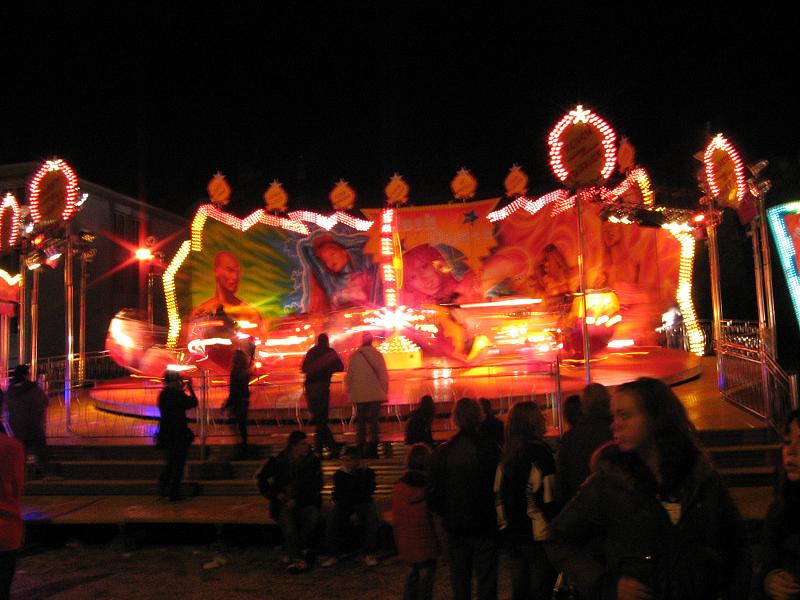This is a full-color nighttime photograph taken outdoors at an exhibition or carnival, capturing a vibrant and lively atmosphere. The focal point of the image is a round, brightly lit stage, which could easily be mistaken for a Las Vegas attraction due to its dazzling display. The stage features a colorful array of lights in green, red, and blue, with a backdrop adorned with large, possibly painted or photographed faces of people. The lights around the stage are very bright and slightly blurry, suggesting motion and energy that permeates the scene. 

This entertaining space requires visitors to ascend a few steps, with a gate positioned in front of it. People can be seen walking up to and around the stage, some standing and observing, while others sit or line up nearby, likely waiting for their turn to experience the attraction. The overall image is slightly grainy and distorted due to the motion of the ride and the low light conditions, adding to the dynamic and bustling feel of the environment. Many of the people in the photograph are wearing jackets, indicating a cooler night. The scene vividly captures a moment of anticipation and enjoyment in a festive setting.